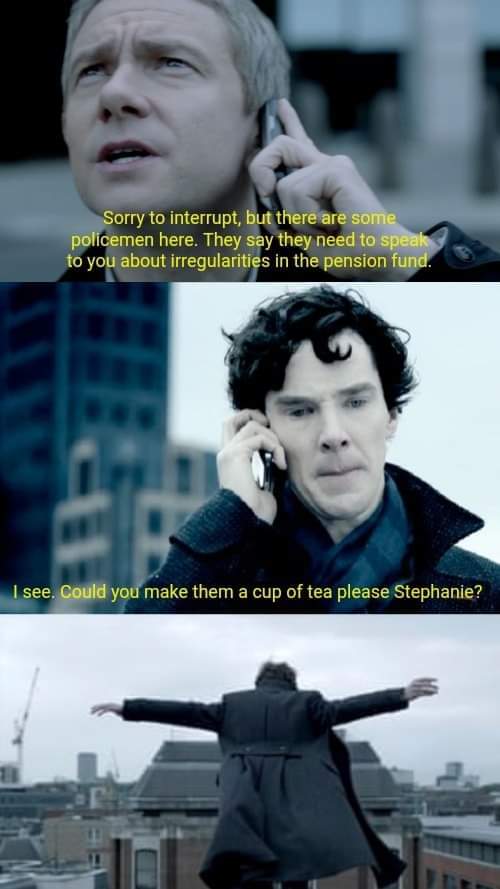This vertical rectangular image appears to be a meme, composed of three distinct scenes from an unidentified movie. The top scene features a man with short gray hair, dressed in a black coat. He holds a cell phone to his left ear with his left hand, his eyes looking upwards. Yellow text at the bottom of this scene reads, "Sorry to interrupt, but there are some policemen here. They say they need to speak to you about irregularities in the pension fund."

The middle scene shows a different man, characterized by his dark, slightly curly hair and pale complexion. He wears a dark coat with the collar popped and appears to be holding a cell phone to his right ear. The background includes a gray sky and several buildings, with skyscrapers visible. This scene also has yellow text at the bottom that says, "I see. Could you make them a cup of tea, please, Stephanie?"

The bottom scene likely features the same man from the middle image but seen from behind. He is wearing a long trench coat and appears to be leaping from a building with his arms outstretched, giving the impression that he’s trying to fly. The background shows various buildings, a crane on the left, and what might be a stadium in front.

Together, these images and captions create a narrative sequence, possibly humorous or dramatic, typical of a meme format.